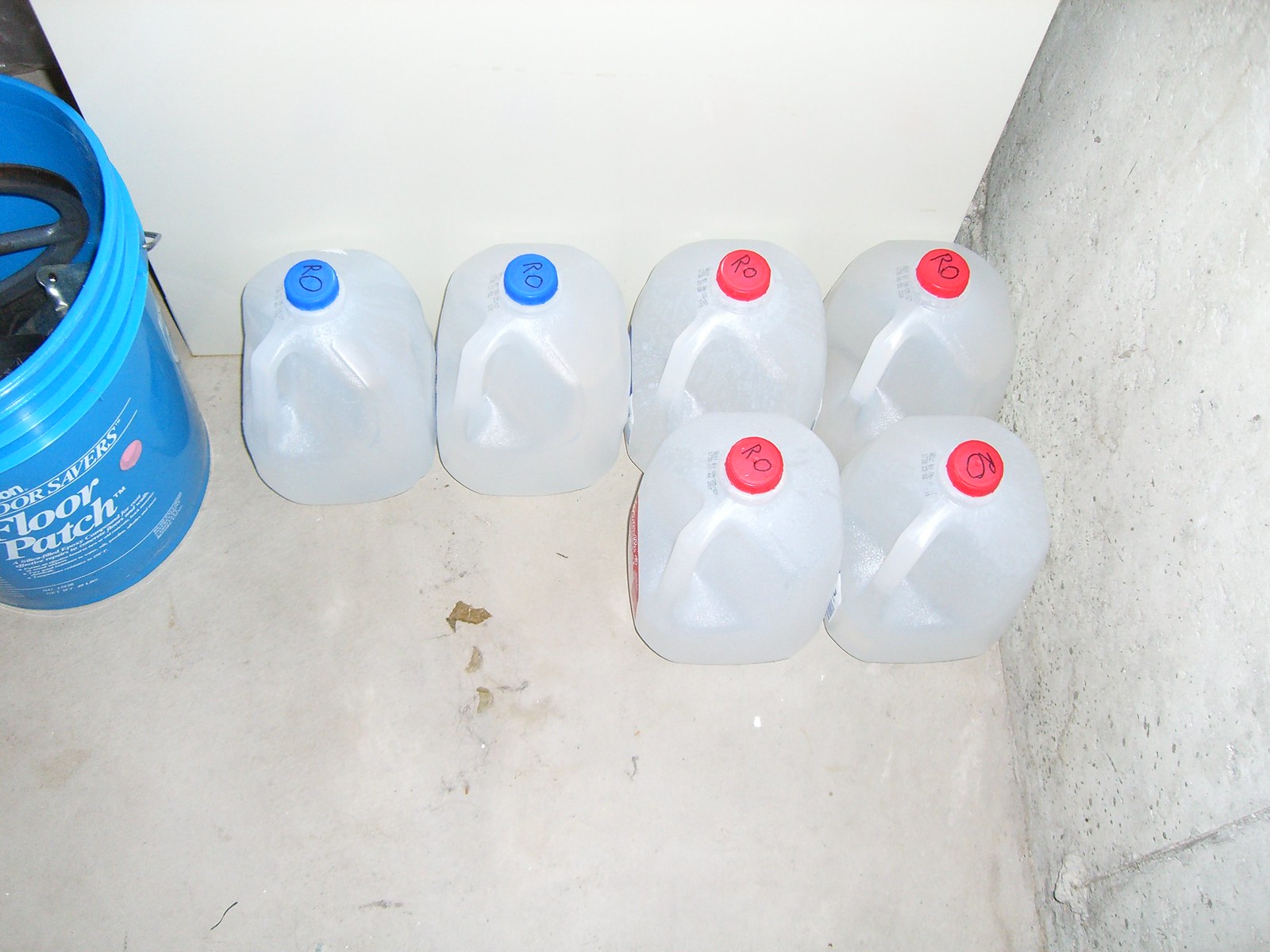This is an overhead view of a corner in what appears to be a basement or garage storage room. The scene features six clear, empty plastic milk jugs positioned against two intersecting walls. The back wall, composed of white wood, extends across the top of the image and meets a white concrete wall that runs vertically. The white flooring, concrete in nature, shows some stains and debris.

In the left side of the image, half of a blue bucket is visible, bearing white text that reads "DOR Savers" and prominently "Floor Patch" beneath it. The bucket appears to contain something black, possibly tools or implements. The six milk jugs are arranged with two rows: the first row against the wall has two jugs with blue caps labeled "RO" in black letters, and four jugs in front of them, two feature blue caps with "RO" markings as well. All jugs seem to be empty and cleaned.

Overall, the image conveys a neat but utilitarian storage setup, highlighted by the contrasting caps and organizational use of space.